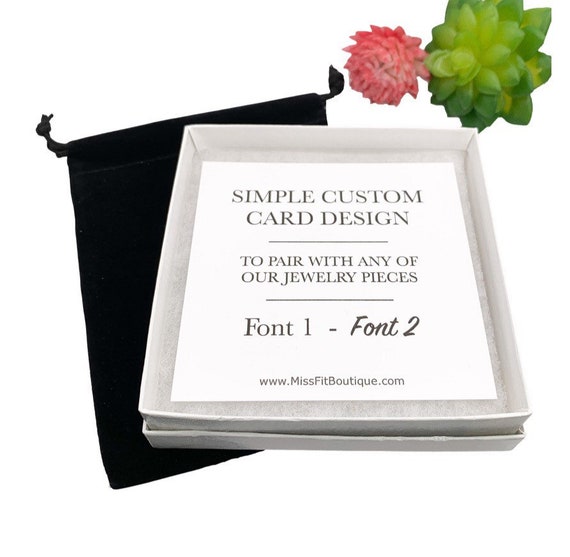The image depicts a silver-colored frame or gift box placed atop a black drawstring bag. At the center, there's a white card with bold black text that reads, "Simple Custom Card Design to Pair with Any of Our Jewelry Pieces. Font 1 - Font 2." Below this text, the website "www.misfitboutique.com" is prominently displayed. The scene includes floral elements in the upper right corner, featuring green and pink petals. The overall color scheme comprises silver, black, white, green, and pink, creating a clean and elegant layout. All objects are neatly arranged in an upright position.